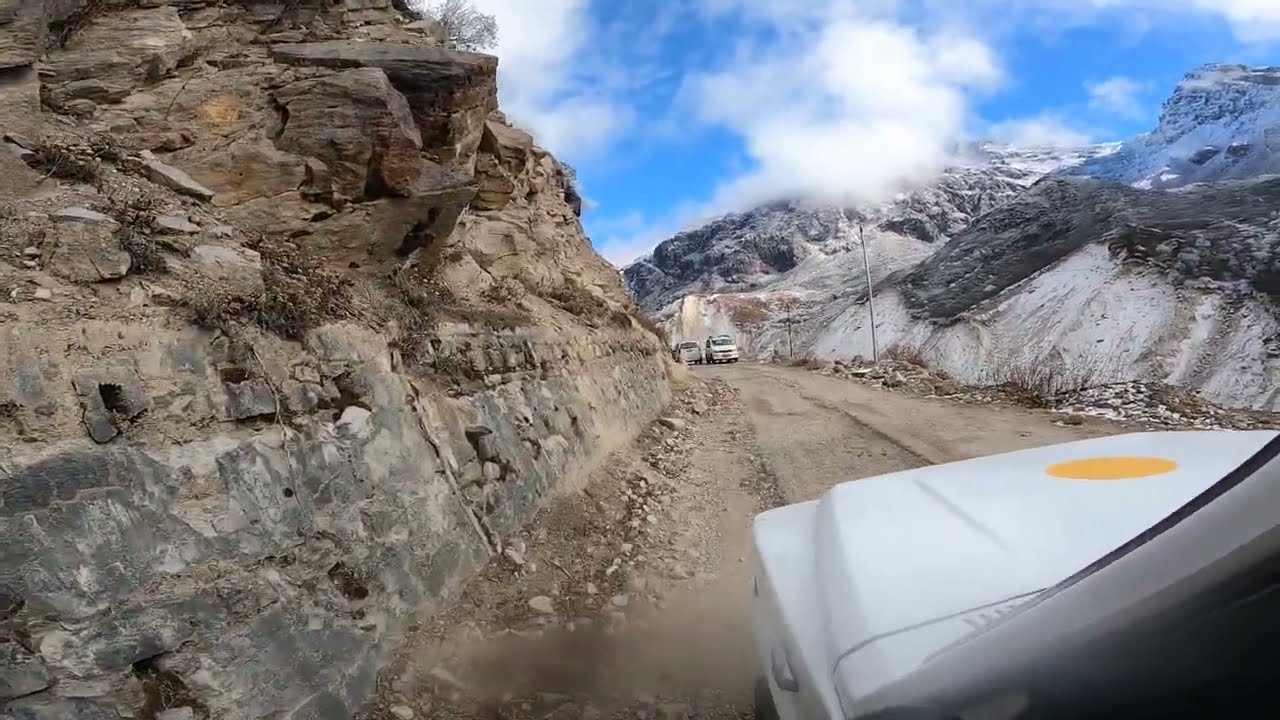This image captures a rugged dirt road carved into the side of a mountain range, exposing jagged rocky peaks on both sides. The perspective suggests the viewer is hanging outside the driver's side window of a white, boxy vehicle, marked by a distinctive bright yellow circle on its hood. This dirt road, appearing well-worn and extending from the bottom right to the center, curves left and gradually disappears behind mountain ridges. Ahead, a white Jeep is coming toward the viewer, just having been passed by another similar vehicle. The landscape is stark with no trees, featuring rocky bluffs and patches of snow capping the high peaks to the right. The environment appears dry with abundant rocks scattered along the roadside. Above, a clear blue sky dotted with white puffy clouds frames the mountainous terrain, enhancing the sense of altitude and isolation. There is a solitary post up ahead without any utility lines attached, adding to the desolate atmosphere of the scene.